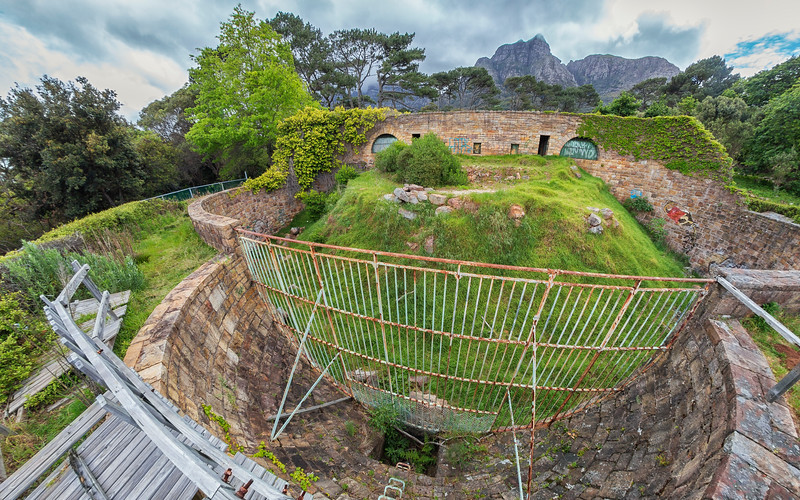The image captures a detailed outdoor scene, reminiscent of an English garden. The focal point is a unique structure that includes a wire basket-like or wire bowl apparatus supported by poles, housing a small hill with bushes atop. Surrounding this central feature are two bowl-shaped structures made of stone bricks in varied shades of brown and cream. Part of the brickwork appears to be overgrown with green vegetation, possibly ivy or moss. In the foreground, there is a rusty white fence and a wooden railing, with a small wooden structure nestled in the bottom left corner. The background reveals a lush, grassy area with different shades of green trees, set against a distant mountain range under a blue sky dotted with white clouds. The fisheye lens effect adds a sense of depth and curvature to the sprawling backyard garden.